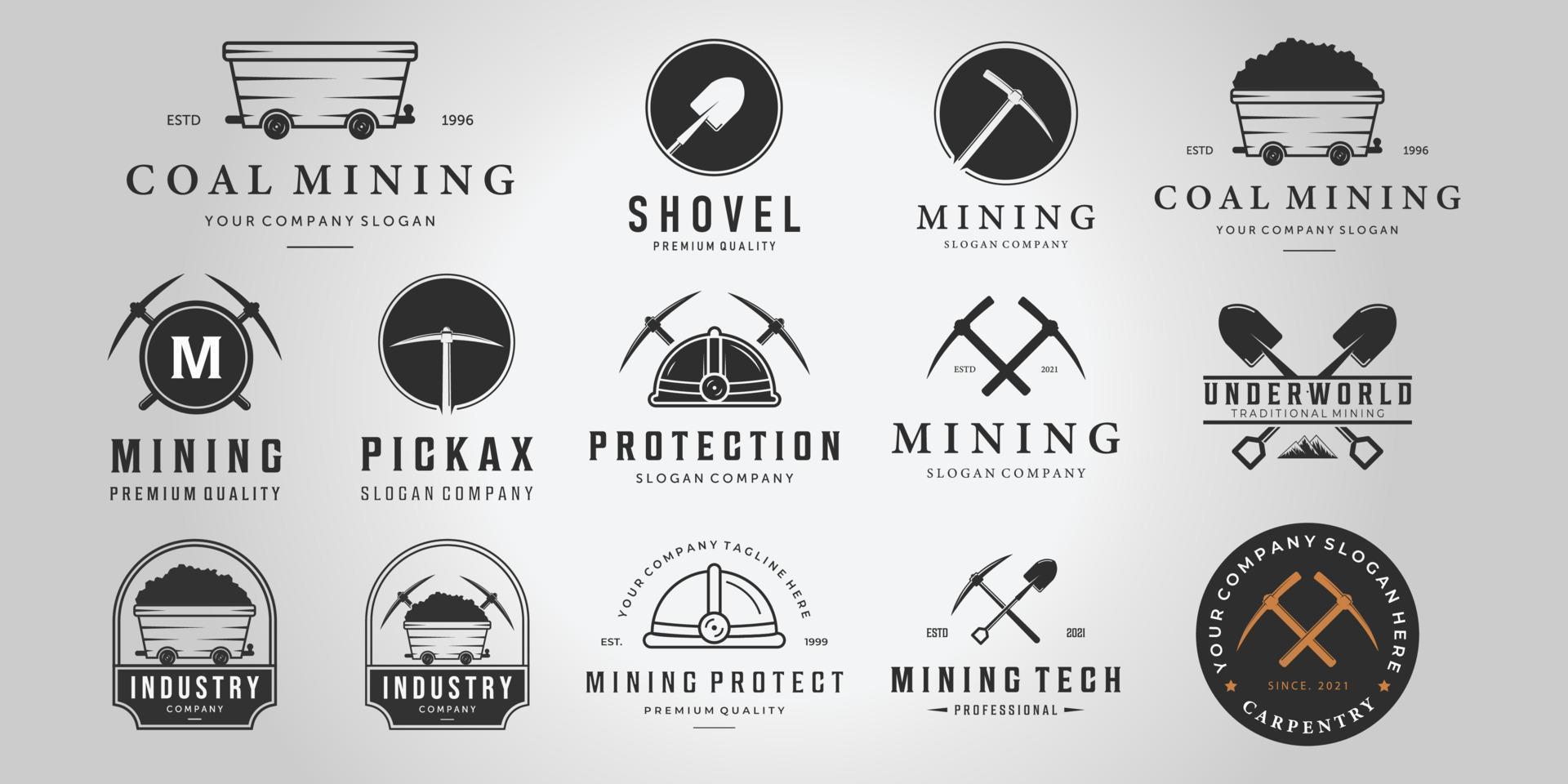This image showcases an assortment of monochromatic digital logos, primarily associated with the mining industry, displayed on a gradient background transitioning from white to light gray. The logos are organized into three rows, with four in the top row, five in the center, and five in the bottom row.

In the top left, there is a logo featuring a mine cart labeled "Coal Mining," accompanied by the phrase "Your Company Slogan" beneath it. The cart is adorned with "ESTD" on the left and "1996" on the right. Beside it, a shovel encased in a black circle reads "Shovel Premium Quality." Next is a pickaxe within a circle, captioned "Mining Slogan Company." To the far right, a similar "Coal Mining" cart logo, this time containing coal, is present with the same slogan.

The center row starts with a circular logo featuring a large white "M" backed by crossed pickaxes and the text "Mining Premium Quality." Next is a white pickaxe in a black circle, labeled "Pickaxe Slogan Company." Following this, a mining helmet with an attached lamp is depicted with crossed pickaxes and the caption "Protection Slogan Company." Further along are crossed black pickaxes stating "Established 2021" and "Mining Slogan Company" below. To the far right, crossed shovels with mountains below and the text "Underworld Traditional Mining."

In the bottom row, a coal cart inside a badge reads "Industry Company," flanked by a coal cart with crossed pickaxes and the same "Industry Company" text. Next is a mining helmet with "Your Company Tagline Here" in an arc above it, flanked by "Established 1999" and "Mining Protect" and "Premium Quality" below. Adjacent is a crossed shovel and pickaxe reading "Established 2021 Mining Tech Professional." The final image, and the only one with color, consists of two bronze pickaxes within a black circle that reads "Industry Company Slogan Here" and "Carpentry," completed with "Since 2021" in the center.